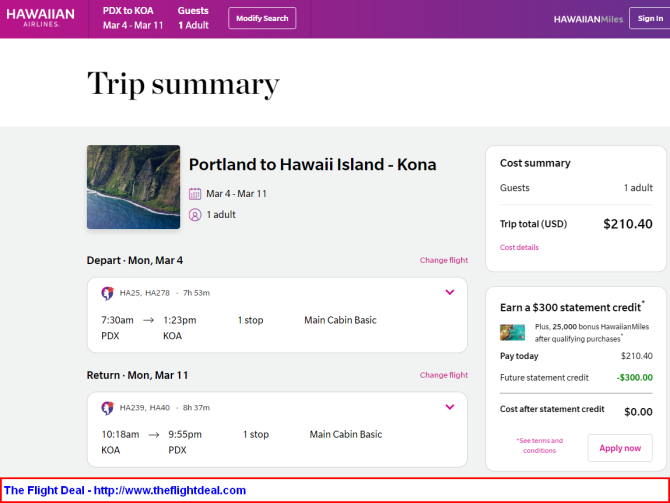The screenshot depicts the Hawaiian Airlines website, prominently featuring a colorful banner that transitions from pink on the left to purple on the right at the top of the page. At the header, a search bar allows users to specify travel details, with options to modify the search as needed. A login option is also available.

The search parameters in the image indicate a flight booking from Portland International Airport (PDX) to Kona International Airport (KOA) on the Island of Hawaii. The travel dates are set from March 4th to March 11th, for one adult passenger. This information is clearly displayed as a visual reminder beneath the search bar.

Below the search summary, there is a detailed trip summary confirming the itinerary. The summary specifies that the journey will be from Portland (PDX) to Kona (KOA) with departure on Monday, March 4th, and return on Monday, March 11th. The traveler has selected the Main Cabin Basic fare option. The total cost for this round-trip flight is $210.40.